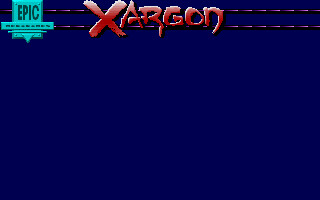This image is a horizontally rectangular screenshot seemingly taken from a video game. The background is predominantly a very dark blue, creating a stark contrast with the elements in the foreground. 

In the upper portion of the frame, two horizontal red dotted lines stretch across the image. On the left side, positioned above these red lines, is a teal-colored square with the word "Epic" distinctly written inside it, suggesting it may be a label or a status indicator within the game. 

Centrally positioned and layered over the red dotted lines is the word "Zargon," written in bold red letters. The unconventional spelling, X-A-R-G-O-N, stands out prominently against the dark background, potentially indicating a significant character, location, or title within the video game's context. These elements are the focal point of this otherwise minimalistic screenshot, suggesting their importance in the gaming scenario depicted.